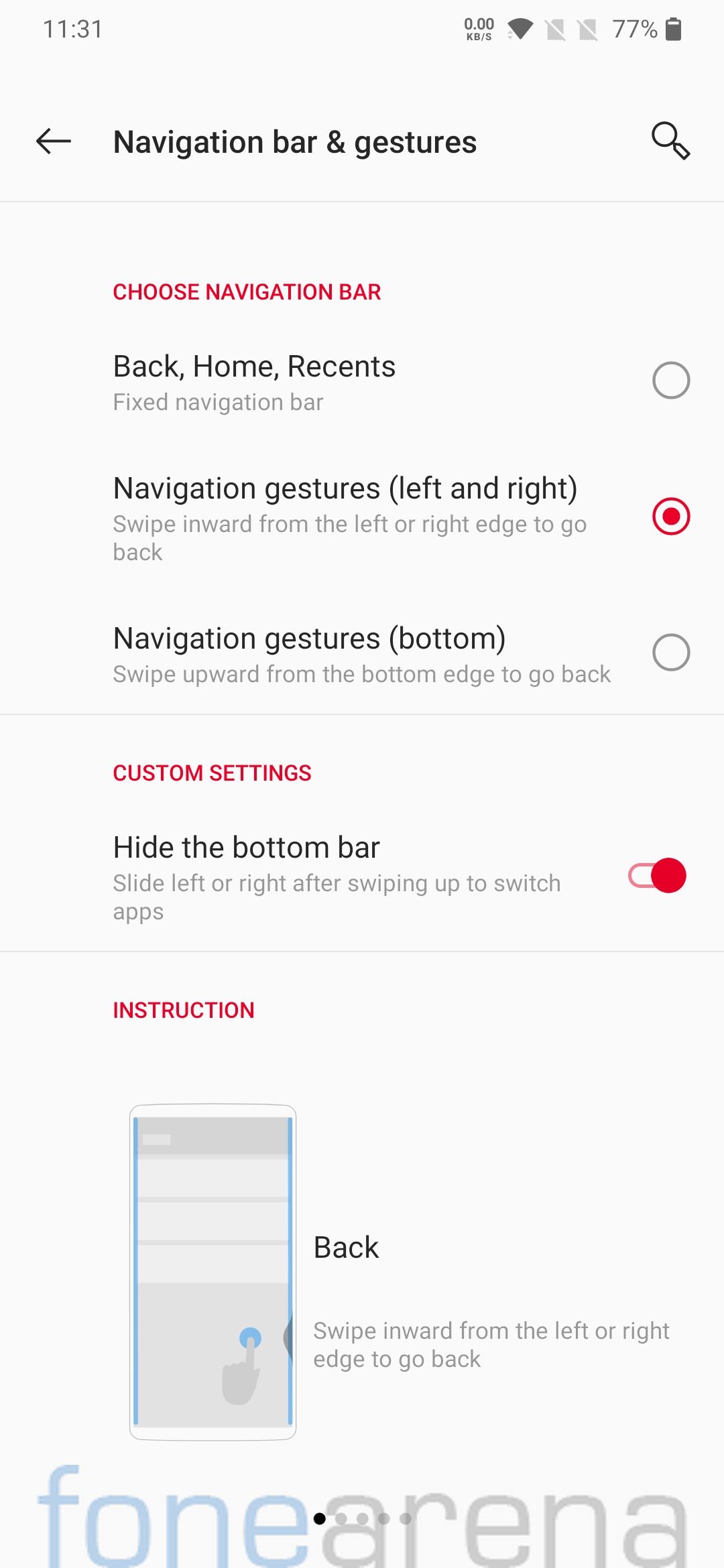The image depicts a smartphone screen with several interface elements and navigational instructions. The battery level is at 77%, and the time shows 11:31. At the top, there is a navigation bar featuring an arrow pointing left and a magnifying glass on the right.

The screen is primarily focused on navigation settings. The phrase "Choose Navigation Mode" is highlighted in red. Below this, various navigation options are listed, including "Back," "Home," "Recents," "Fix Navigation Bar," and "Navigation Gestures." Instructions for each option detail how they function. For instance, navigating back can be achieved by swiping inward from the left or right edge. 

One specific navigation gesture is emphasized with a red circle, indicating that this setting is currently active. This setting, "Swipe Upward from the Bottom Edge to Go Back," is detailed with further customization options, such as "Custom Settings," which are also highlighted in red. It provides additional tips, like hiding the bottom bar and sliding left or right after swiping up to switch apps. A toggle bar nearby is shown to be turned on, enabling these custom settings.

The bottom section of the screen includes an instruction area allowing users to interact with the navigation. The terms "Phone," "Arena," and "Fone" appear, accompanied by a series of five circles, where the first circle is black, indicating the current selection, and the remaining circles are gray.

This detailed layout provides comprehensive navigation instructions and settings customization for the smartphone user.